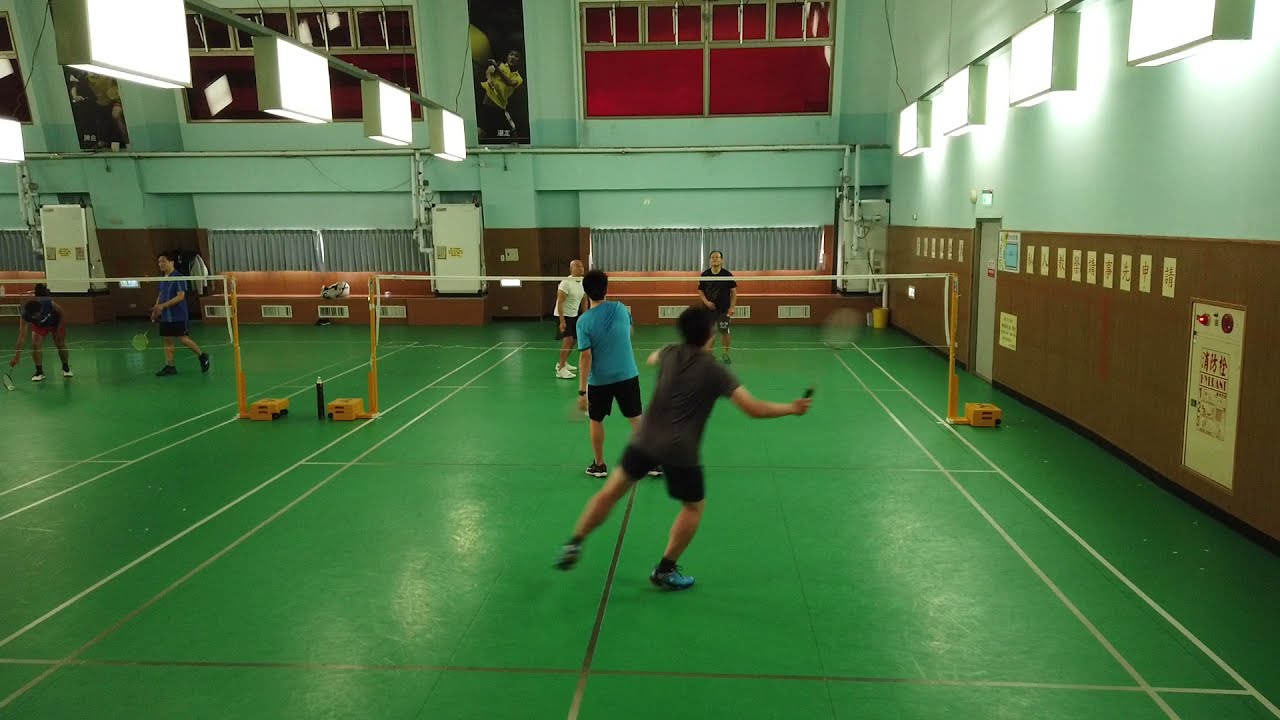In this image, a group of people are actively engaged in racket sports within an indoor facility. The venue features two adjacent courts, each surfaced with dark green flooring marked by vertical lines. The indoor setting is confirmed by the presence of enclosing walls, which are brown on the bottom and transition to white towards the top, adding to the venue's vintage ambiance. Square-shaped lights hang down from the walls and the ceiling, ensuring the facility is well-illuminated.

On the right court, four individuals are clearly visible, divided into two teams. One player, centered in the image, is poised to hit a ball, wearing a brown shirt, shorts, and shoes. This player’s partner, who stands nearby, is clad in a light blue shirt and black shorts. Their opponents comprise a player in black on the right and another in a cream-colored yellow shirt on the left.

The left court is partially visible, showing two more players. One, wearing a blue shirt, is slightly bent over, while the other in a black shirt, is walking to the left. Both courts are separated by nets that are supported by orange posts, which add a noticeable detail to the setting.

The facility's walls are adorned with various posters and banners, some depicting athletes, and there are small yellow and red signs on the brown section of the walls. Additionally, there is a red window located in the upper part of the building, towards the middle and left side. Despite the suggestion by one caption that the sport might be badminton, the overall description suggests that the participants are more likely engaged in tennis or paddle ball, given the presence of the net and rackets.